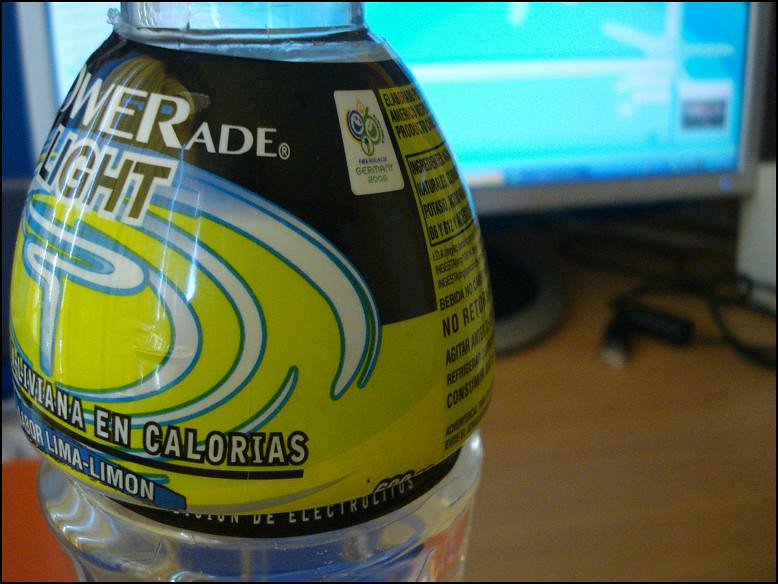This image captures a close-up of a Powerade Light bottle, likely lemon-lime flavored, inferred from the "LIMA-LIMON" wording in Spanish on the label. The bottle, made of clear plastic with a yellow and black label, partially obscures the "Powerade" logo, showing only "W-E-R-Ade." The text on the label includes nutrition facts and mentions "calorias" and "electrolytos," indicative of a Latin American region. In the background, a computer monitor with a bright blue display featuring stars and lines is visible. This set-up is complemented by a tangle of black cords and a USB cable resting on a light wooden desk. The monitor, edged in a silver frame with a blue LED at the bottom right, provides a modern technological touch to the scene.